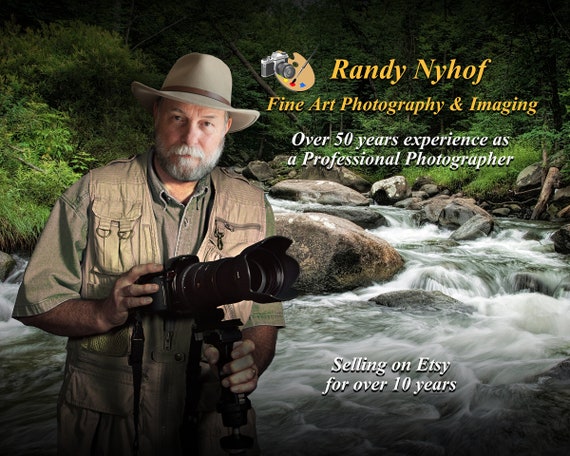The photograph is an advertisement featuring Randy Nighhoff, a seasoned professional photographer with over 50 years of experience and more than a decade of selling on Etsy. The majority of the background is dominated by an exhilarating scene of a whitewater creek surrounded by abundant greenery, with turbulent water cascading over numerous rocks. Randy Nighhoff, a serious-looking Caucasian man, stands confidently in the foreground, clad in a safari outfit consisting of a tan vest and a tan brimmed hat. He holds a large black camera with an impressive lens. The text over the image, presented in bold italic Times New Roman font, reads: "Randy Nighhoff, Fine Art Photography and Imaging. Over 50 Years of Experience as a Professional Photographer. Selling on Etsy for Over 10 Years."